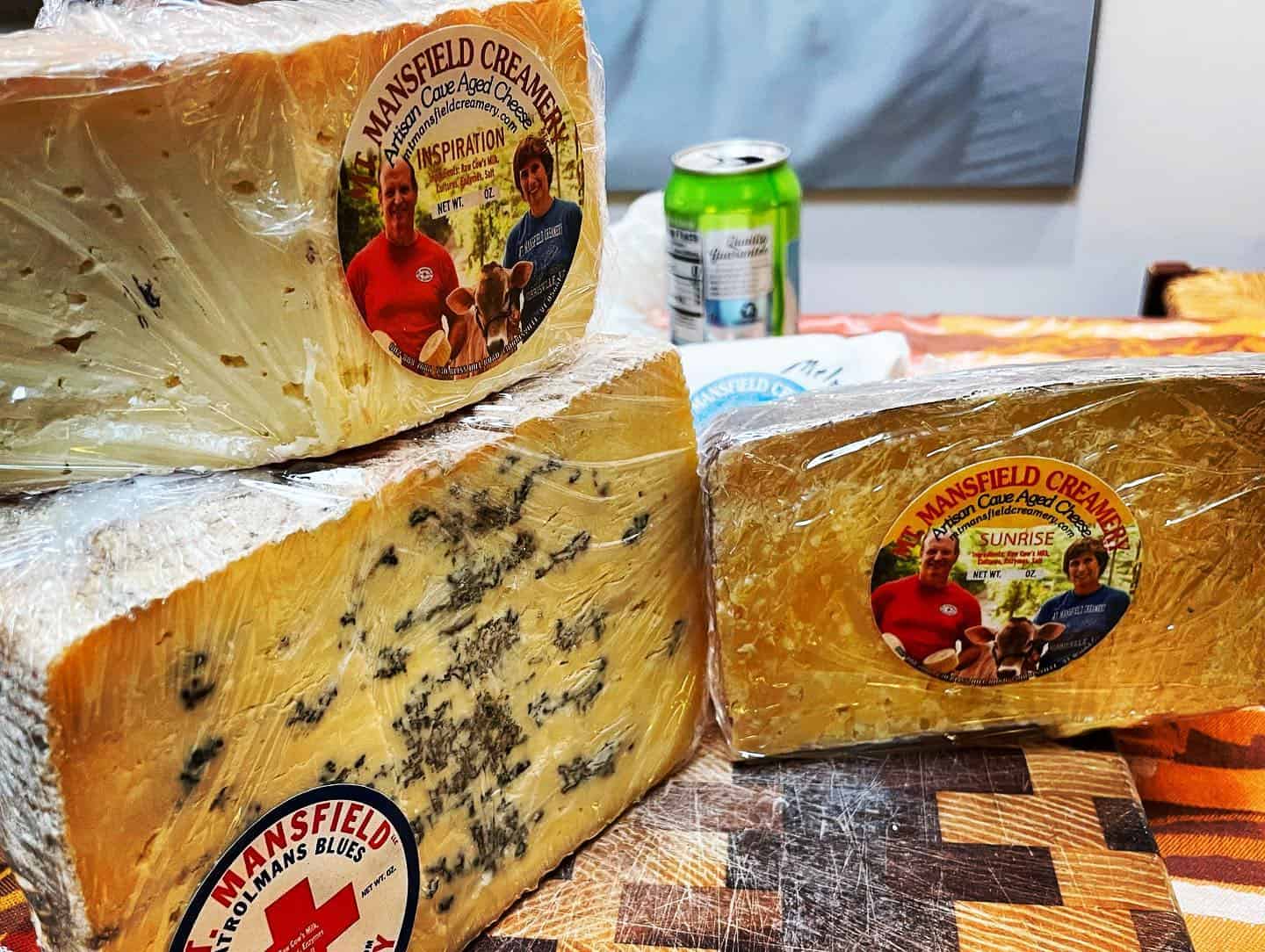This detailed close-up photograph features three blocks of cheese wrapped in clear plastic, prominently displaying labels from Mansfield Creamery. The labels read "Artisan Cave Aged Cheese" and feature a smiling man in a red t-shirt on the left, a woman in a blue t-shirt on the right, and a donkey at the center. Two blocks of cheese are stacked on top of each other on the left, with another block positioned to the right. The checkerboard table, composed of varying shades of brown, supports the arrangement. In the blurry background, a greenish-yellow soda can with an open tab sits next to a dark gray screen, adding depth to the composition.